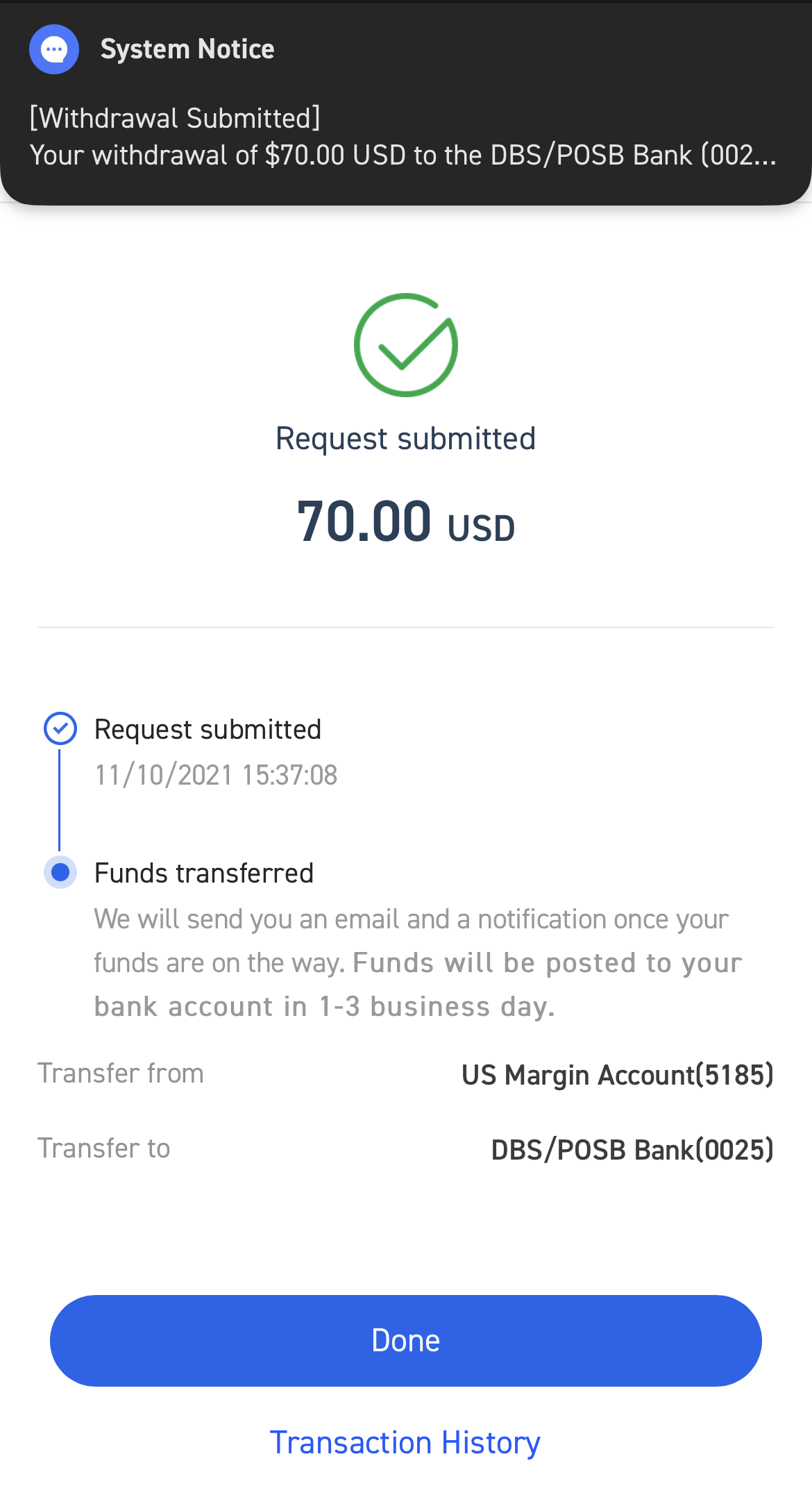**Screenshot of Transaction Confirmation Dialogue**

At the top, there is a black system notice with a small blue circle containing an ellipsis. It displays the message:

**[Withdrawal Submitted]**

Your withdrawal of $70.00 USD to the DBS POSB Bank (ending in 002...) 

Below that, a green check mark inside a green circle appears, accompanied by the message:

**Request Submitted**

Further below, the amount:

**70.00 USD** 

is displayed in bold. A horizontal line separates this information from the section below.

Next, there is a blue circle with a blue check mark and the following text:

**Request Submitted**  
*11 Oct 2021, 15:37:08*

Following that, another blue circle, this time solid in the middle, contains the message:

**Funds Transferred**  
*We will send you an email and a notification once your funds are on the way. Funds will be posted to your bank account in one to three business days.*

(Note: 'business day' is incorrectly written in singular form)

Below, the transfer details are listed:

- **Transfer from:** US Margin Account (ending in 5185)
- **Transfer to:** DBS/POSB Bank (ending in 5025)

At the bottom, there is a prominent blue 'Done' button.